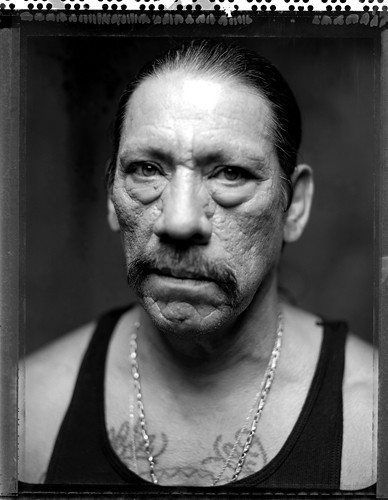This tall, rectangular black and white photograph features a rugged man with light skin, appearing to be of Hispanic or Mexican descent, visible from the shoulders up. His weathered face is marked by prominent wrinkles, deep bags under his eyes, and a scattering of scars, suggesting a history of many battles, possibly in boxing or other tough engagements. The man is adorned with a thick, drooping mustache and has slicked-back black hair that reveals both of his ears, which might appear slightly disfigured, adding to his hardened look. He wears a black tank top with thin straps, partially concealing a tattoo on his chest. Around his neck are two necklaces, with one chain standing out as thicker and shinier than the other. His large nose and the light reflecting off the center of his forehead accentuate his serious expression and tough demeanor. The dark background enhances his formidable presence, evoking the image of a seasoned actor often cast in villainous or tough-guy roles in numerous films.